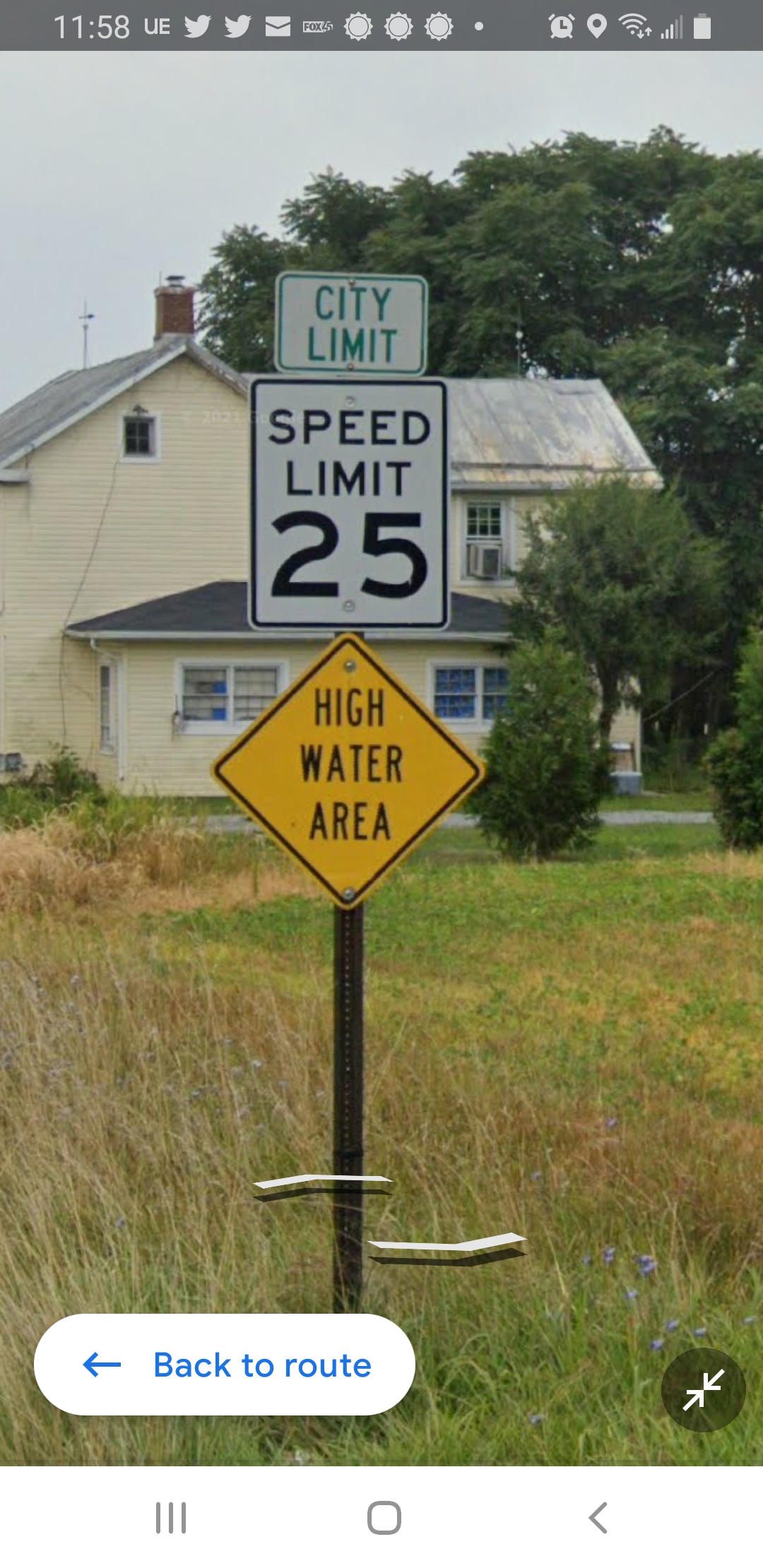This image is a screenshot from a Maps app on a smartphone, depicting a detailed street scene. At the center of the image is a black pole with three attached signs. The top sign is a smaller square with "City Limit" written in green letters on a white background. Below it, there is a larger, rectangular speed limit sign stating "Speed Limit 25" in black letters on a white background. The bottom sign is a yellow diamond shape with "High Water Area" written in black letters. This pole and its signs are centrally placed in the picture, directly in front of a light yellow house that has a roof, brown chimney, and multiple windows. Large trees can be seen behind and in front of the house, casting shade over the scene. The grassy area around the pole and house has both green and brown patches. At the top of the screenshot, typical phone icons are visible, while at the bottom, there is a white label reading "Back to Route" with a left-pointing arrow, indicating navigation directions on the screen.